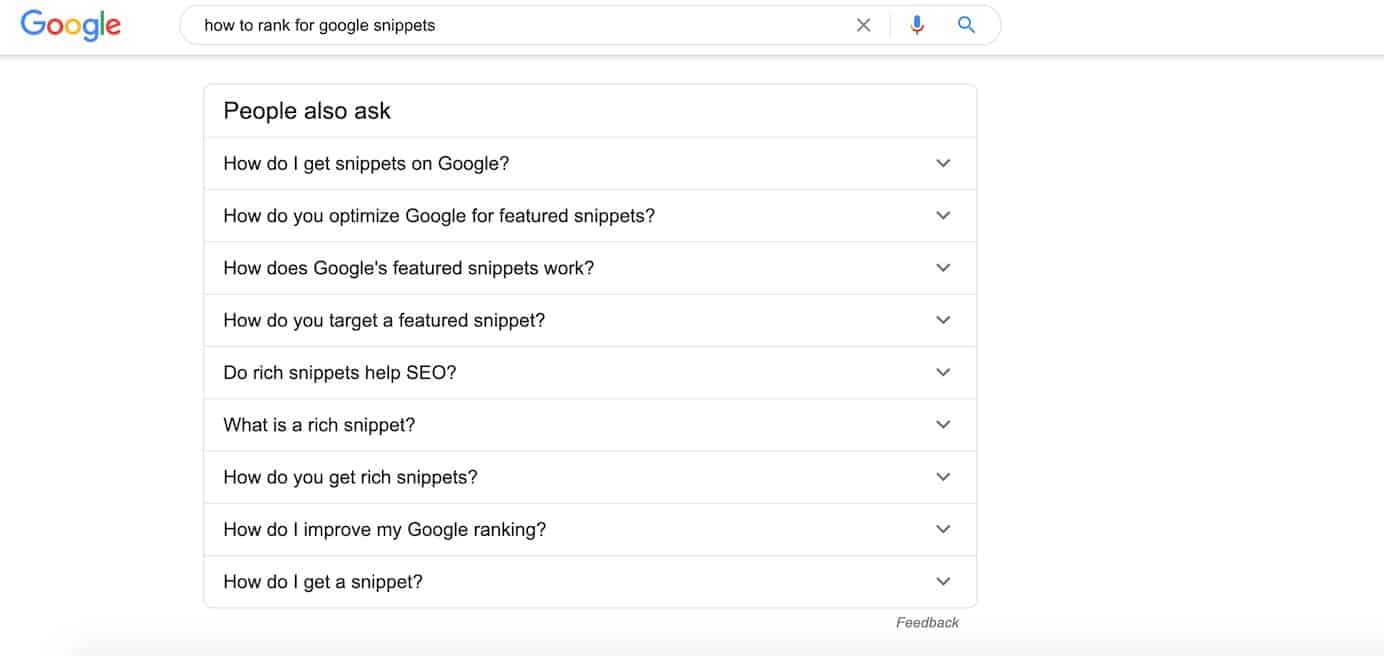This image captures a screenshot of a Google search page focusing on the query "how to rank for Google snippets." The screenshot is in landscape orientation without defined outside borders, giving it an expansive look. At the top, a thin gray border demarcates the header section from the main content area. In the top left corner of the header, the Google logo is prominently displayed, featuring the iconic multi-colored letters—with a blue "G," red "O," yellow "O," blue "G," green "L," and red "E."

The main focus of the image is the white search bar at the top center, filled with the query "how to rank for Google snippets" in black font. Adjacent to the search bar, there are icons for closing the search (an 'X'), a microphone symbol for voice search, and a magnifying glass icon for executing the search.

Below the search bar, the search results section begins, characterized by a clean, white background. The most prominent feature here is a white, square-shaped box with a thin gray border labeled "People also ask." This box presents a series of related questions in black text:

1. How do I get snippets on Google?
2. How do you optimize Google for future snippets?
3. How does Google feature snippets work?
4. How do you target a featured snippet?
5. Do rich snippets help SEO?
6. What is a rich snippet?
7. How do you get rich snippets?
8. How do I improve my Google ranking?
9. How do I get a snippet?

Each question has a drop-down arrow on its left side, allowing users to expand for further information and potentially more detailed explanations. The collection of questions suggests that the individual conducting the search is looking for specific guidance on optimizing their content for Google's featured snippets.